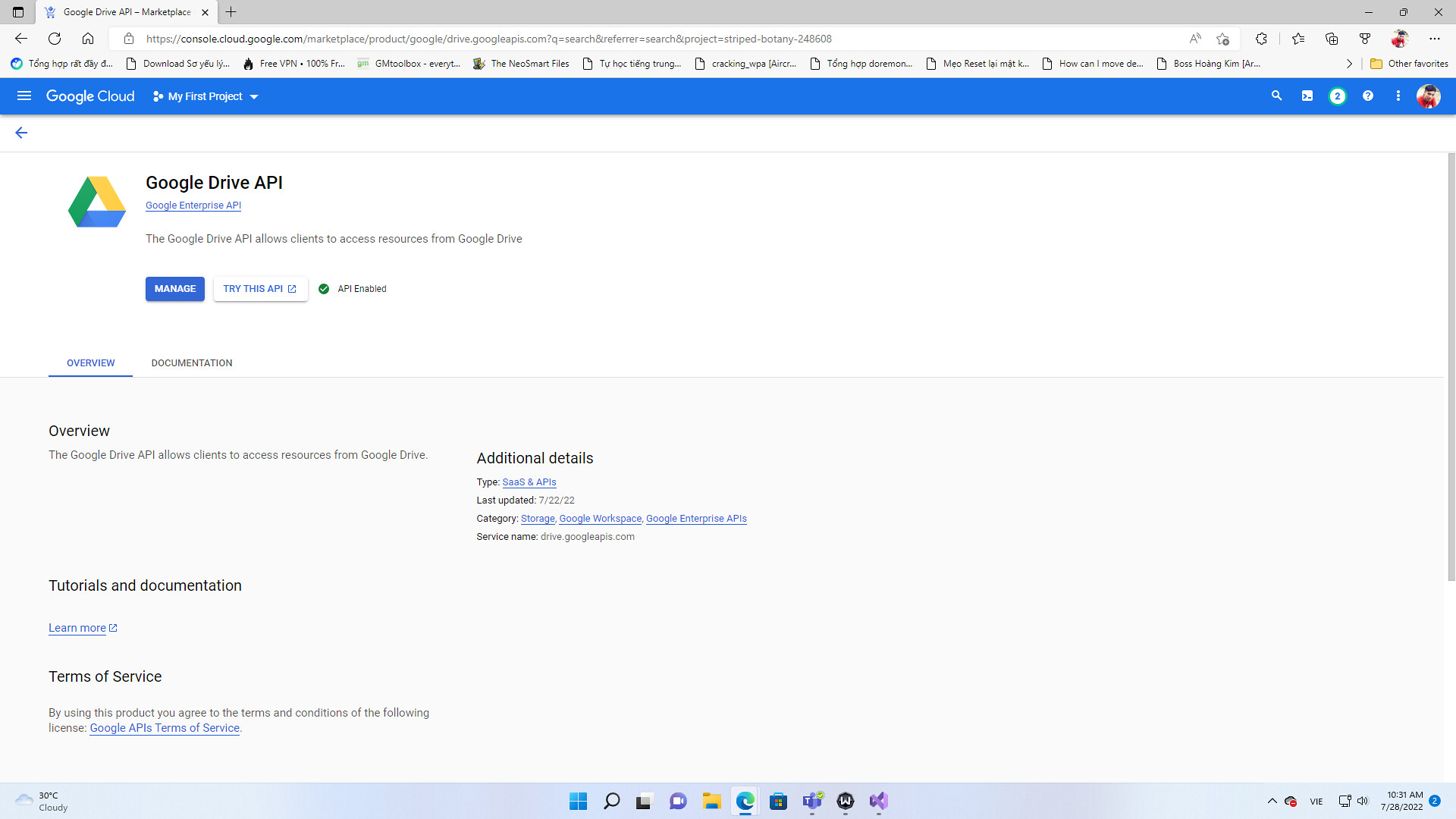This image depicts a browser window open to the Google Developers page, specifically showing details about the Google Drive API. The page has a white background occupying the top third, while the remaining two-thirds are grey. At the very top, in black letters, "Google Drive API" is prominently displayed. Just below, transitioning into the grey section, there's a header titled "Overview," followed by a description explaining that the Google Drive API allows clients to access resources from Google Drive.

Beneath this overview section are various links labeled "Tutorial and Documentation" and "Terms of Service." Additionally, a light blue line spans horizontally across the bottom of the image, indicating several open tabs and clickable options available in the browser.

At the very top of the image, a search input field displays the text that was entered, though it is quite small and difficult to read due to the font size.